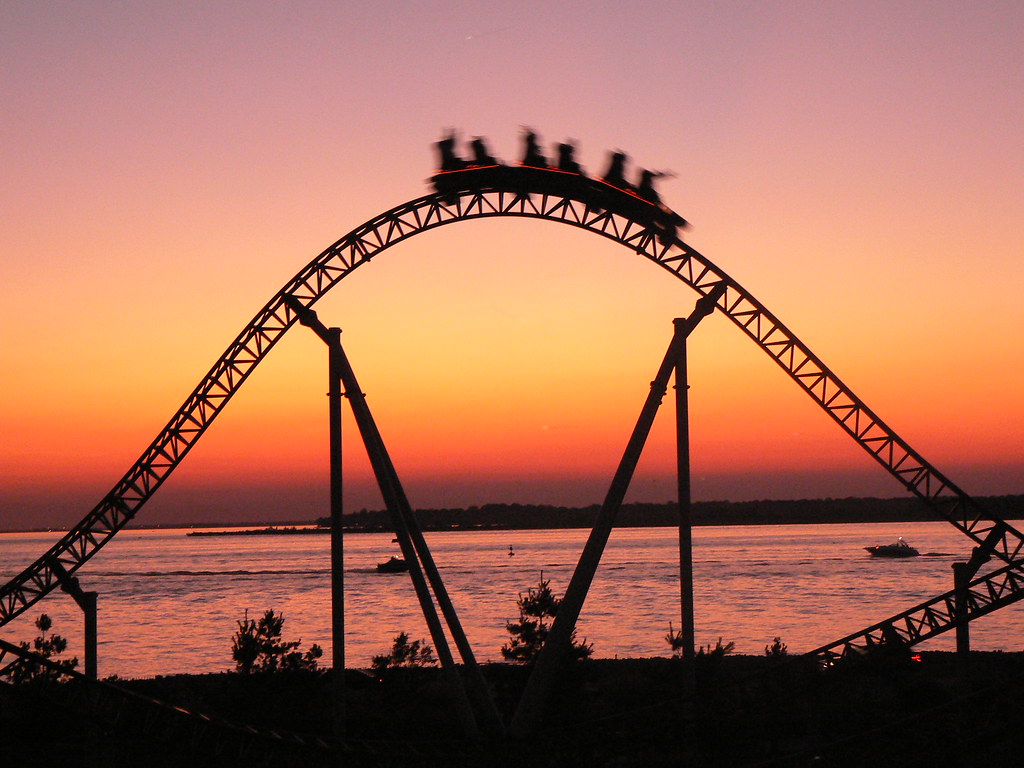This vibrant sunset photograph captures a dramatic outdoor scene featuring the silhouette of a roller coaster with a group of six people riding it, blurred from motion. The roller coaster's curved frame is silhouetted against a stunning sky that transitions from deep purple to pink, orange, and yellow hues. Below the coaster, the ground shows silhouettes of small trees and bushes. In the background, a large body of water reflects the sky's colors, with two boats visible on its surface, adding to the tranquil yet dynamic atmosphere of the scene.